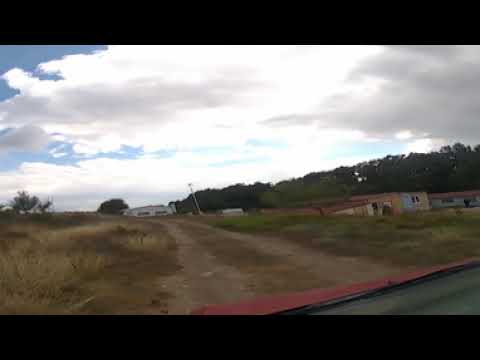The image is a fisheye lens photograph capturing a wide, slightly curved view of a landscape from the back of a red car. The lower half of the image primarily displays brown dirt, stretching from the left side across to the right. The car's rear windshield reflects parts of this ground and the blue sky above, which is interspersed with clouds particularly concentrated on the right. In the lower right corner, some areas of the dirt are tinged with red and gray hues. A chain-link fence runs horizontally from the left side to just past the center of the image, behind which there are additional trees and distant, dark-colored buildings. On the right side of the frame, there's a bushy, lone tree with a line of other trees extending towards the middle of the image, contributing to a sense of depth and perspective.